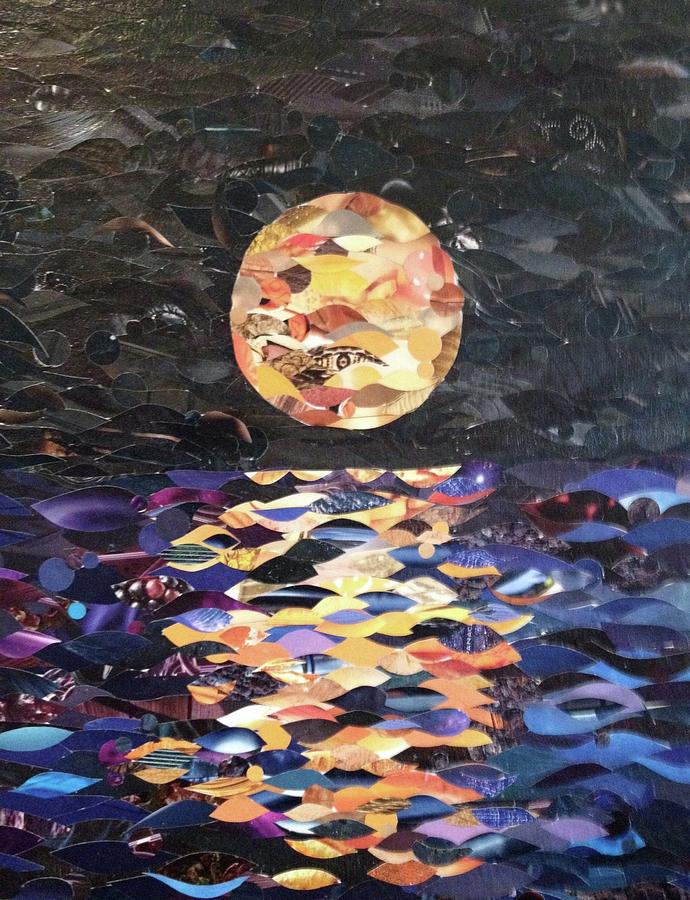This abstract, modern painting in portrait mode features a round shape at the top, reminiscent of either the moon or the sun, cast against a black sky. This celestial body is composed of various vibrant hues of yellow, orange, red, peach, and brown, forming a mosaic-like pattern of oval and crystalized shapes. The lower portion of the artwork portrays a sea or ocean, depicted with hues of blue, purple, and indigo, suggesting nighttime waters. Scattered within this blue expanse are multicolored shapes, possibly representing fish swimming in different directions or the reflection of the celestial body above. This artistic piece invites personal interpretation, blending elements of both a serene night sky and a tranquil sea in a complex, detailed, and colorful fashion.